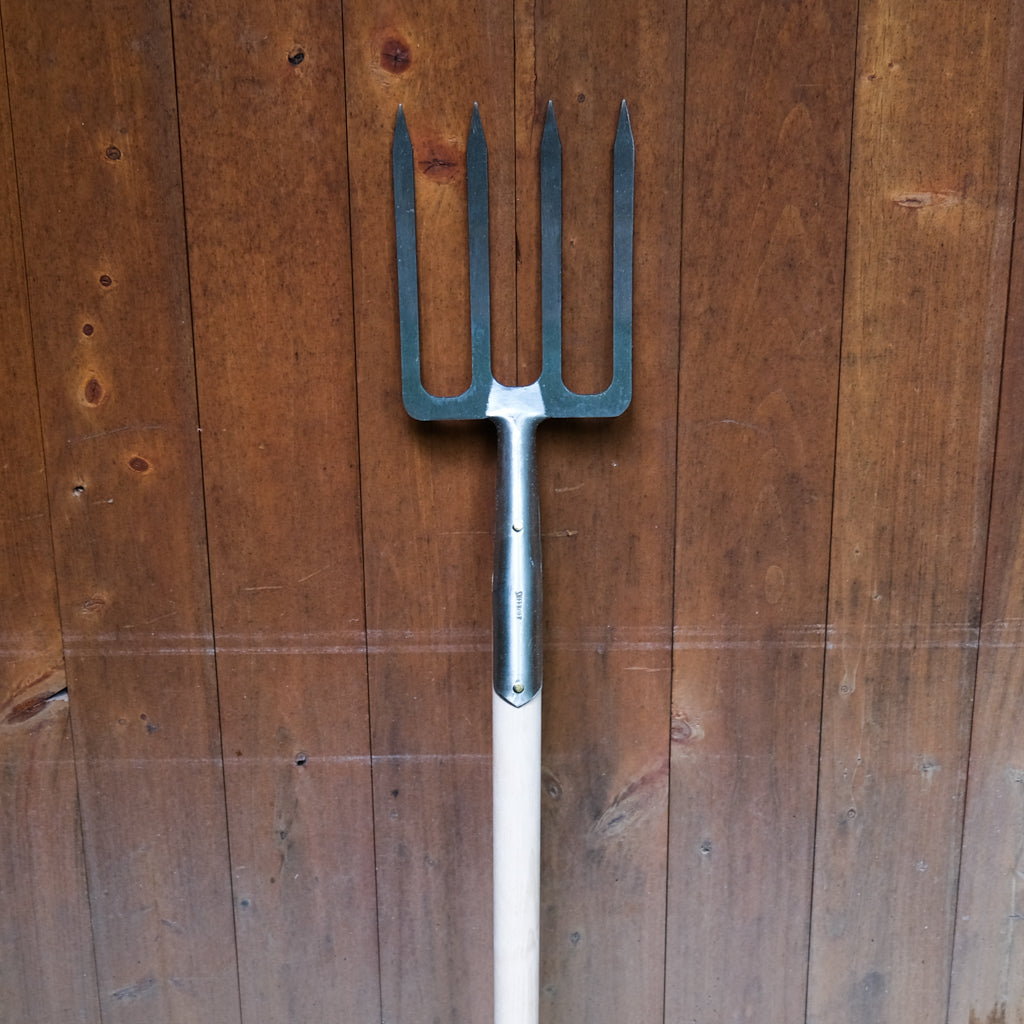In the center of this photograph, a small pitchfork-like item with four metallic tines and a white handle is prominently featured, leaning against a richly hued dark brown wooden wall. The tool’s handle is positioned at the bottom with the silver and black metal tines at the top, showcasing a square-shaped outer edge. The background consists of hardwood panels with visible imperfections and drag marks, suggesting previous movement of furniture. The wall’s texture varies from dark brown to a more ashen color closer to the bottom, giving it a distinctive, weathered appearance. The simplicity and clarity of the image emphasize the contrast between the sleek, metallic pitchfork and the rustic, wooden surface behind it.